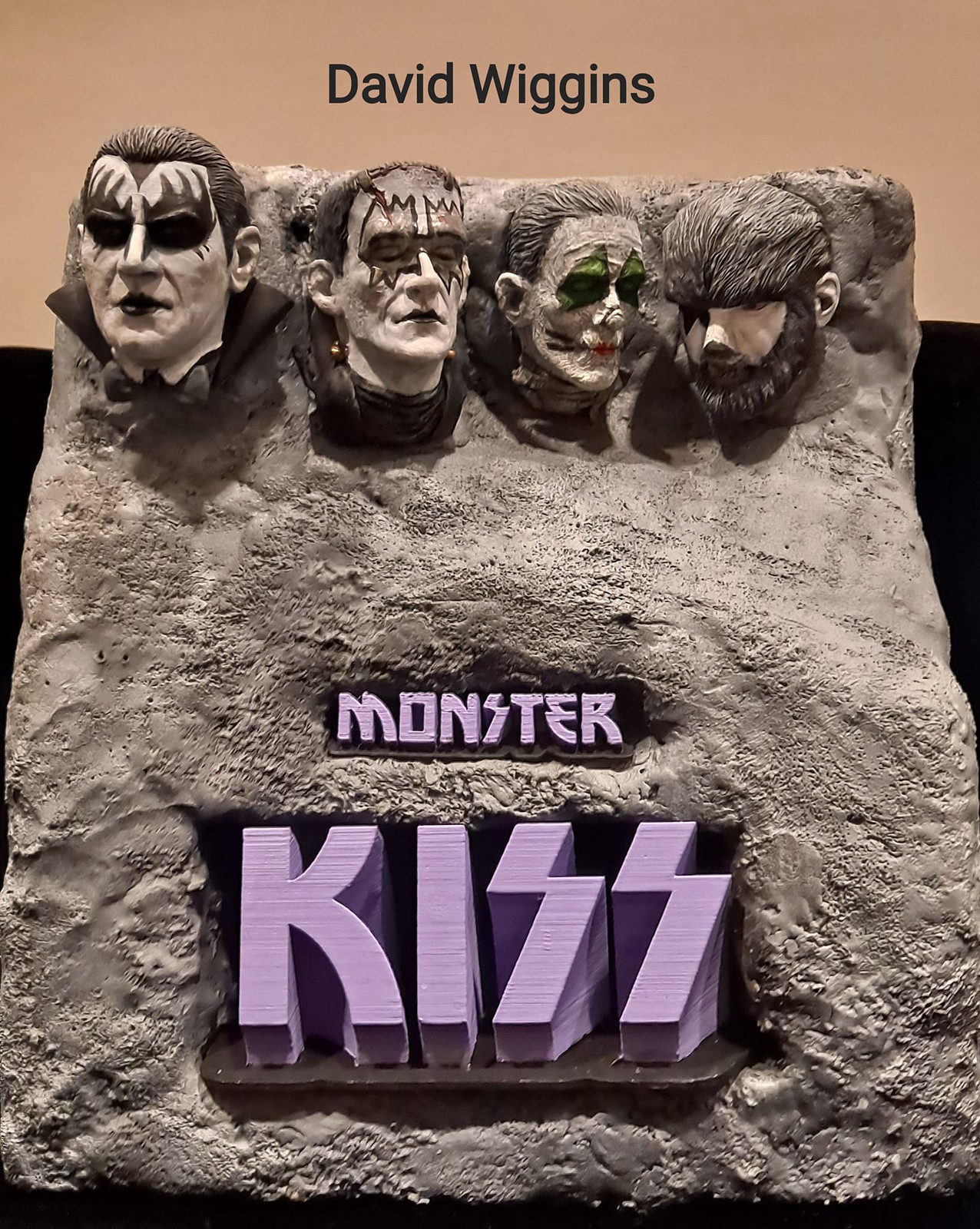This image is a digital illustration, possibly done in Photoshop, depicting a parody of Mount Rushmore with the faces of the four KISS band members instead of the presidents. The sculpture is set against a light gray rocky background and a black backdrop, with a light brown section at the top where "David Wiggins" is written in black text. The heads of the KISS members protrude from the top of the rocky structure, each adorned with their signature black and white makeup. The far left head resembles a Dracula-like figure with a high-pointed black collar and a widow's peak. Next is a Frankenstein-like face with KISS-style face paint, followed by a head with cat-like whiskers and markings. The far right head appears to be a werewolf with a thick mane of hair and a long beard. Below the sculpted heads, in large light purple text, it says "Monster" followed by "KISS" with the iconic "SS" depicted as thunderbolts.